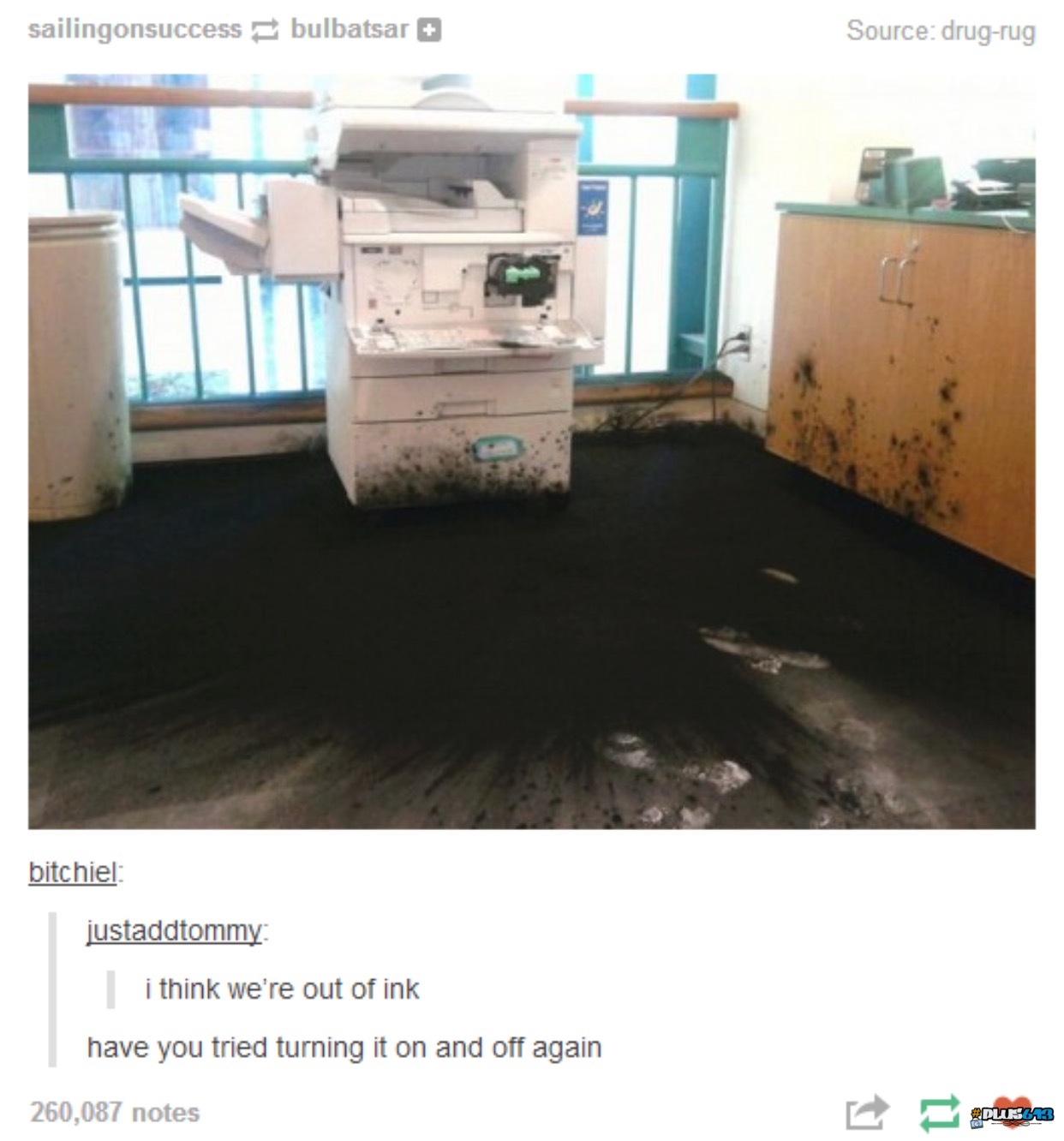In the image, a white office copier is positioned in front of a window or an open area, revealing a green balcony railing in the background. Surrounding the copier, the floor is covered in a cloud of spilled toner, emphasizing that this printer uses a powdery substance rather than liquid ink. The toner has also coated the bottom of the copier and partially dusted the adjacent brown wooden cabinet.

Above the copier, blue text reads "sailing on success, full Batsar," followed by a symbol of a plus, potentially denoting a user or status. Additionally, the number of notes on the image is quite high, reaching 260,087. One user named BITCHEL comments at the bottom, saying, "I think we're out of ink," to which another user, Just Add Tommy, replies, "Have you tried turning it on and off again?" This dialogue is part of the humorous meme presented by the image, highlighting the toner mishap in a light-hearted manner.